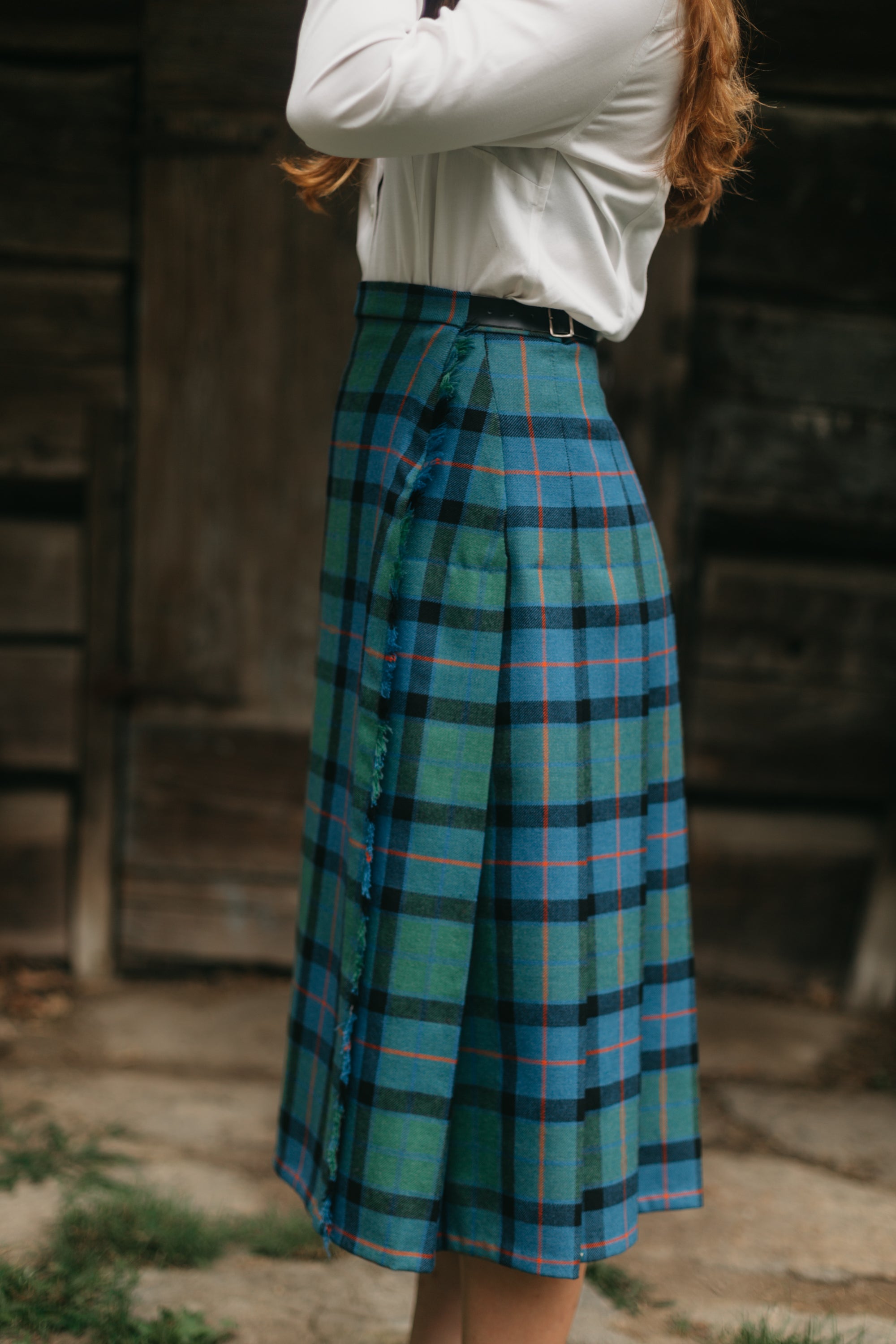The image captures a woman standing sideways, viewed from her shoulders down to her lower legs. She is dressed in a white long-sleeved button-up shirt, paired with a long checkered dress that features a mix of dark blue, light green, and light blue background adorned with thin black horizontal lines and thinner vertical lines in shades of red and orange. The dress has a sophisticated flip on the front and is accentuated by a black belt with a silver lock at the back. The skirt portion of the dress extends from just above the belly button down to her shins. She is positioned in front of a wooden building, possibly a barn, with a ground surface scattered with dirt and small patches of grass.